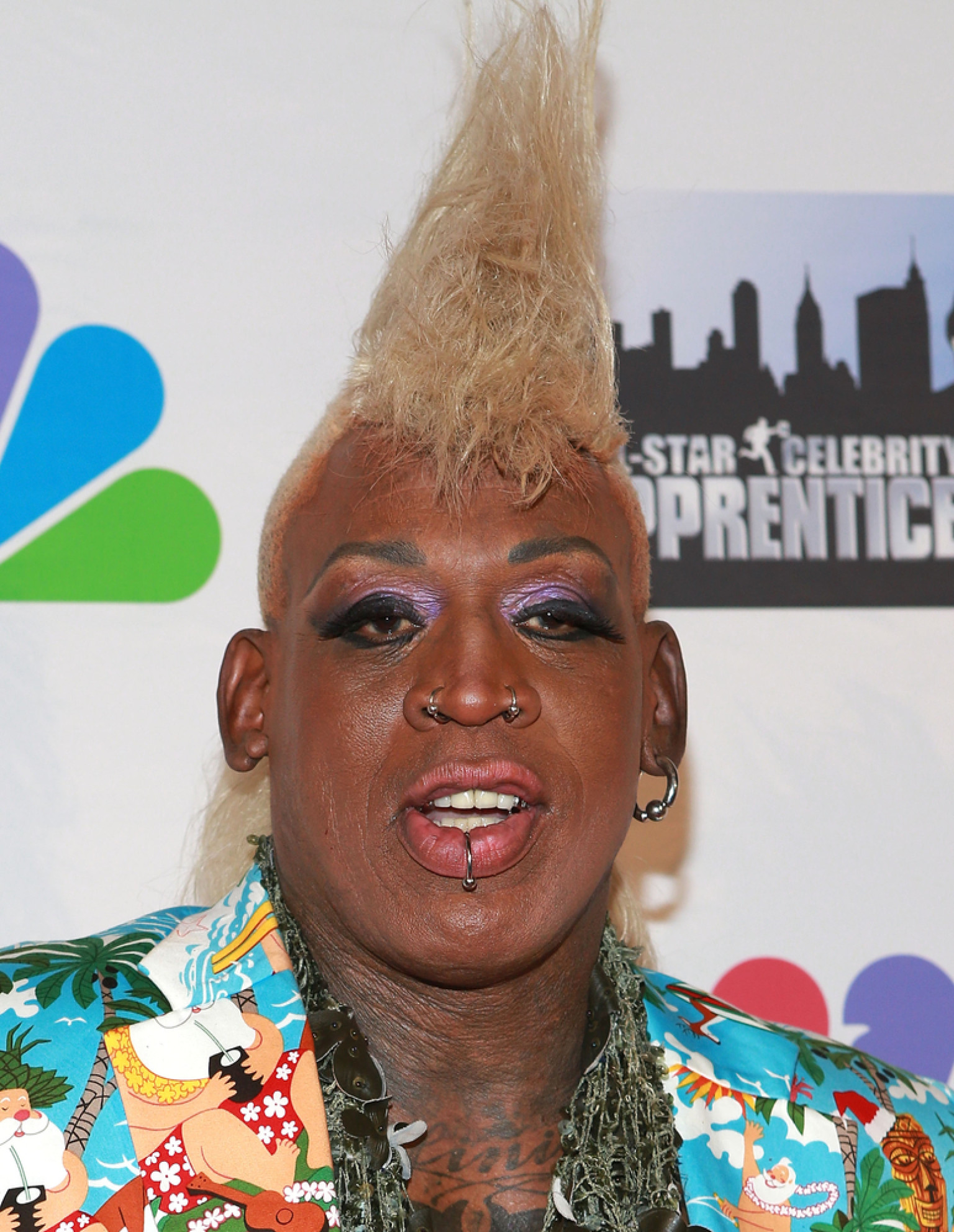The photograph depicts Dennis Rodman at a press conference, distinguished by his striking appearance. His blonde mohawk rises dramatically, higher than typical, giving a wild flair to his look. Rodman's face is adorned with various piercings: two nose rings, a large earring, a hook ring earring, and a lip ring. Enhanced with makeup, he sports purple eyeshadow, mascara, eyeliner, and peachy lip color. His dark skin and oval-shaped face provide a strong contrast to his flamboyant attire—a multi-colored Hawaiian blazer featuring red, green, blue, gold, and palm trees, complemented by a green shirt with various designs. His numerous tattoos are visible, stretching from his chest to his neck. Behind him is a white wall with signage, including an NBC logo on the upper left and an "All-Star Celebrity Apprentice" poster on the upper right, indicating the event's theme.